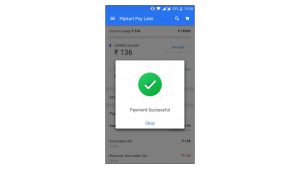The image depicts a cell phone screen showing a payment confirmation interface. At the top of the screen, there's a blue strip displaying various icons, including vibrate mode, Wi-Fi connection, and cell signal bars. Due to the low resolution of the image, details are somewhat blurred when enlarged.

In the middle section, the text "136₹" (Indian rupees) is visible, suggesting that this amount is being referenced or processed. Below this text, there is a gray-tinted area that might contain more details but is obscured by the poor image quality.

On the surface layer of the screen, a prominent white square featuring a green circle with a white checkmark inside indicates a successful transaction. Beneath this icon, the text appears to confirm "Payment Succeeded" with an "OK" button below it.

The primary colors visible in the image include blue, white, black, gray, and green. The overall context and exact details remain somewhat unclear due to the image's blurriness, but the general impression is that the screen is showing a successful payment transaction involving 136 Indian rupees.